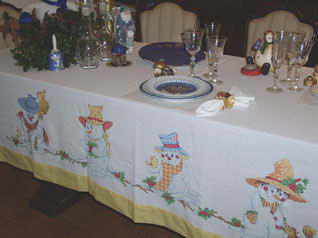The photograph captures a festively decorated wooden table with a broad base, partly visible beneath a white tablecloth adorned with a charming snowman pattern and a yellow border. The snowmen are illustrated wearing various rustic costumes, including hats and scarves, and seem to be arranged in a lively winter scene. The top of the tablecloth is plain white. The table is set with colorful dishware, including a white china plate with a blue rim and a central circular design, alongside a solid blue plate. These are complemented by elegant, stemmed wine glasses arranged in groups of three. The table also features a decorative centerpiece that resembles a wreath, alongside a stand-up snowman and a Santa statue dressed curiously in a blue outfit. Surrounding the table are ornate, padded chairs styled in a French provincial or Baroque fashion. The overall setting evokes a festive, possibly children's dinner scene during the holiday season, with a cozy and whimsical atmosphere accentuated by details like silverware, napkins, and a subtle arrangement of handbills and winter vegetation.